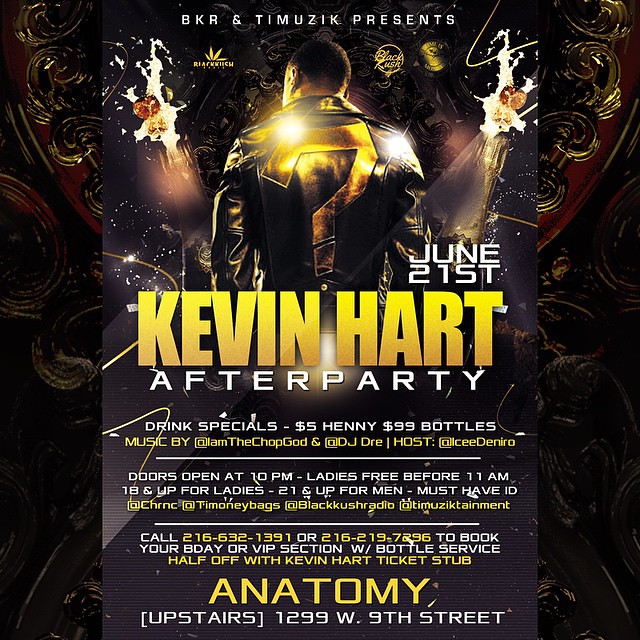The poster is an advertisement for an event titled "Kevin Hart After Party." Prominently featuring a back view of a man—presumably Kevin Hart—wearing an elaborate leather jacket with a large gold question mark, this poster is vibrant and ornate with intricate lighting and shading effects. At the top, it reads, "BKR and Tim Music Present Kevin Hart After Party," followed by the event date, June 21st. In the middle, "Kevin Hart After Party" is displayed in large yellow font. Below, details include various drink specials, such as $5.00 for any drink and $99 bottle deals. The event is to be held at "Anatomy," located at 1299 West 9th Street, with doors opening at 10 PM. Additional information notes that ladies are free before 11 PM and age restrictions apply: 16 and up, or 18 and up for women, and 21 and up for men with ID required. The poster's background is dark but rich with gold highlights, giving it a luxurious and dynamic appearance.